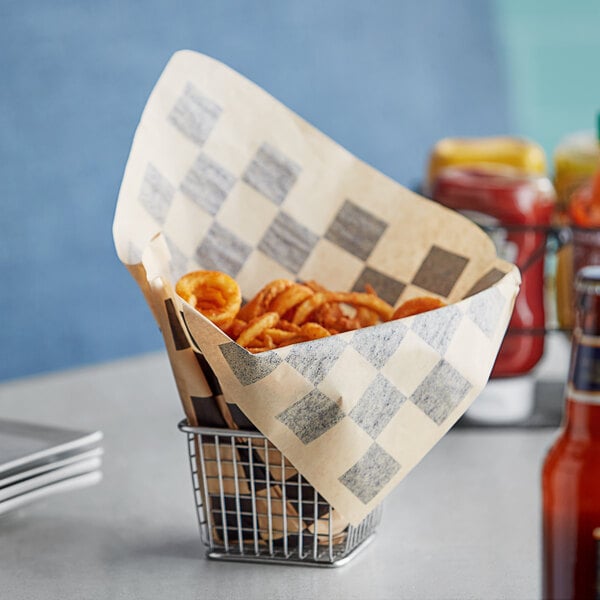A square image depicts a wire metal basket sitting on a white table. The basket is lined with checkered wax paper and overflowing with golden brown curly fries. To the left, a stack of white square plates with blue trim is partially visible by an inch or two. In the bottom right corner, there is a partial view of a bottle of beer, unopened and only about a third of it shown. The background features a blue wall and a condiment rack with a Heinz ketchup bottle and what appears to be a mustard bottle behind the fries. No silverware is visible in the image.